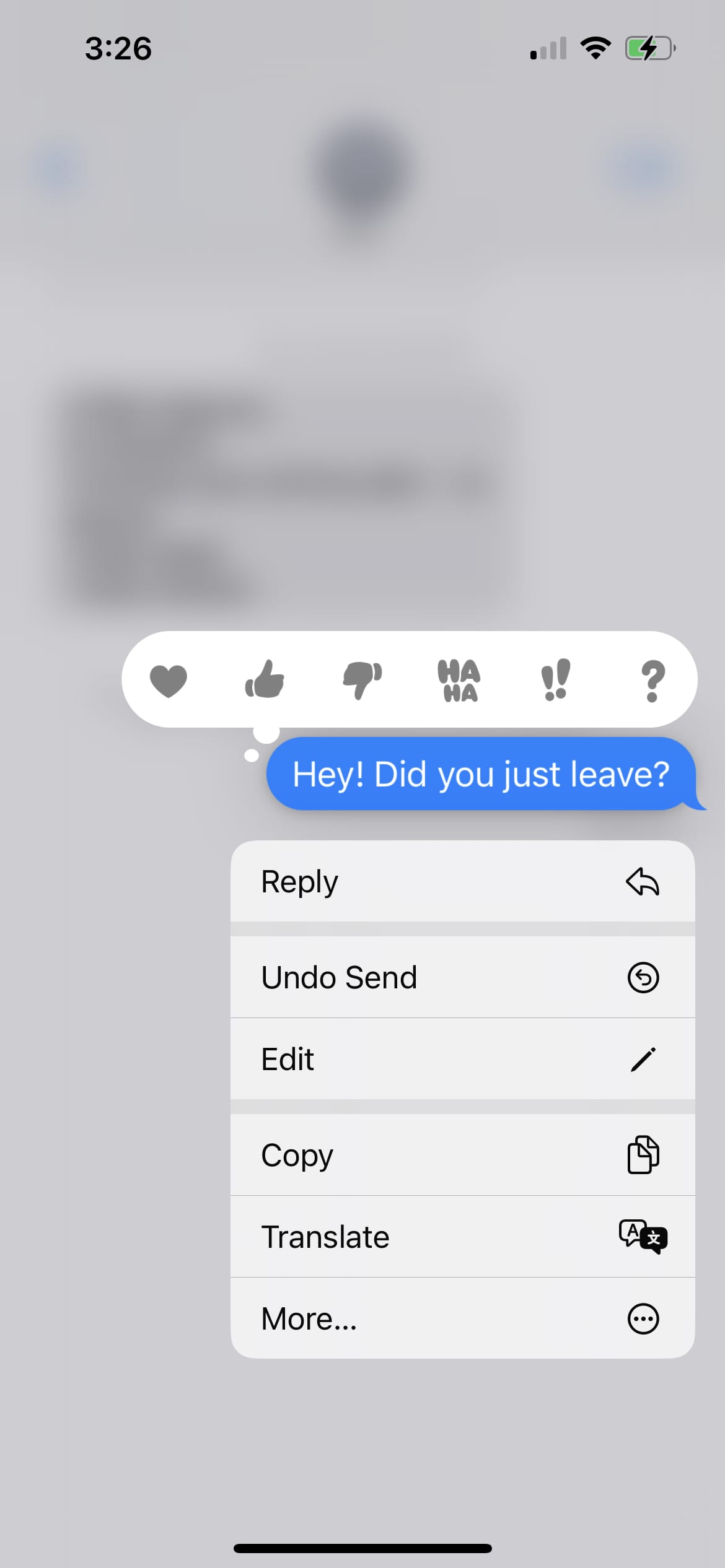The screenshot displays a phone interface with a grayish-purple background. At the top left corner of the screen, the time reads 3:26. Signal indicators are located in the top right corner, showing one bar of cellular reception, full Wi-Fi connectivity, and a battery level at approximately 50%.

Below these status indicators, there is a text message interface. A row of emojis is visible, laid out from left to right including: a heart, a thumbs up, a thumbs down, a laughing face with "ha ha," two exclamation marks, and a question mark.

Directly beneath the emoji row is a blue text box containing the message: "Hey, did you just leave?" Following this, there is a reply option labeled "Reply" with an arrow pointing to the right. Subsequent to this, there are multiple options listed vertically: "Undo Send," "Edit" accompanied by a pencil icon, "Copy," "Translate," and finally, "More." A thin black line is observed at the bottom of the image, signifying the end of the screenshot.